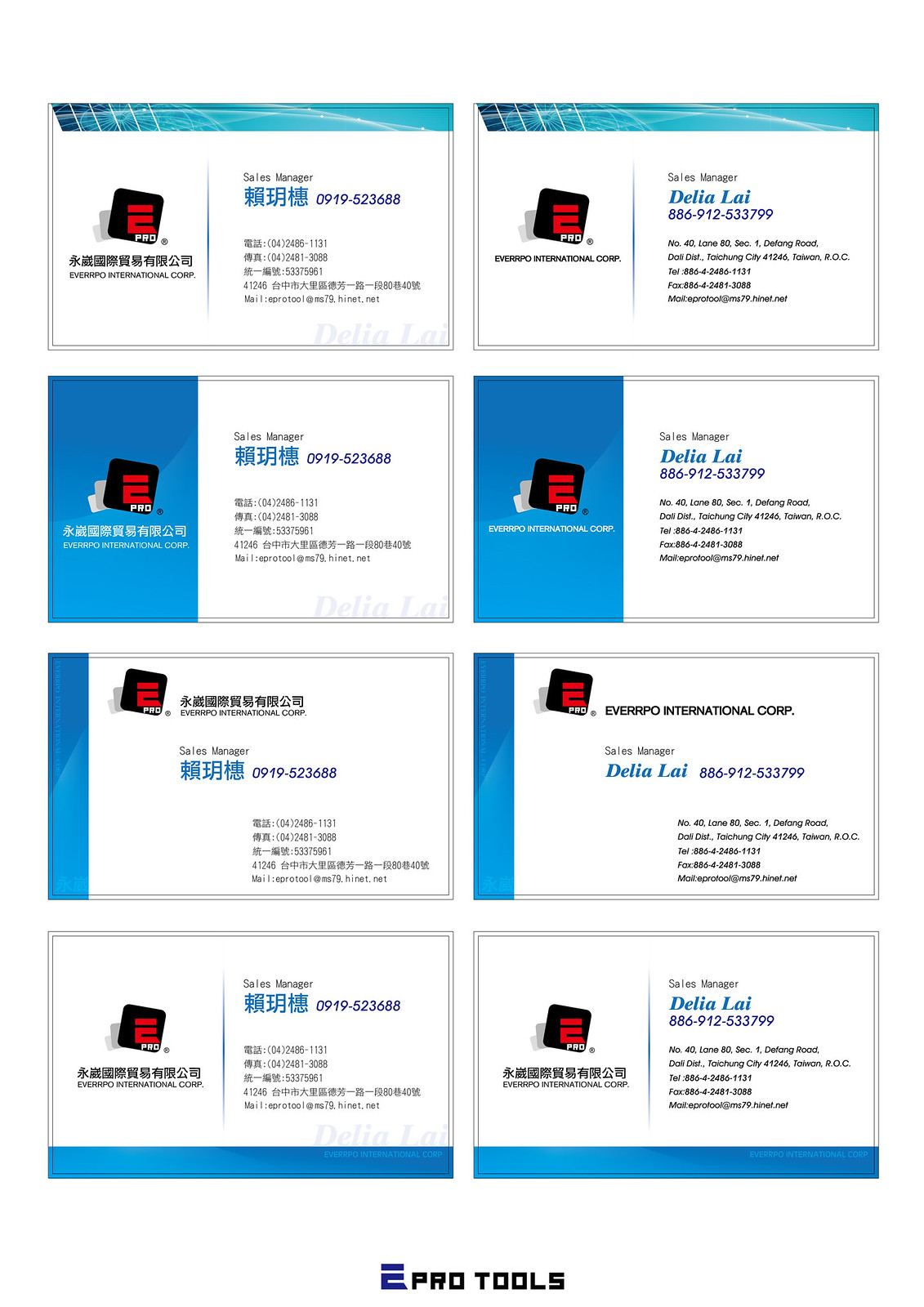The image is a detailed photograph showcasing a collection of eight business cards arranged in a column of four, side by side. Each card represents Delia Lai, the Sales Manager at Everpro International Corp., located in Taiwan. The business cards display variations of similar designs, serving as a sample set for potential custom business card orders. The cards prominently feature contact details, including a phone number (886-912-533-799), the company address (No. 40, Lane 80, Section 1, Defang Road, Dali District, Taichung City, 41246, Taiwan, ROC), a telephone number (886-424-861131), a fax number (886-424-813088), and an email (eprotool@ms79.hinet.net). The text appears in both English and Chinese, possibly along with other languages. At the bottom of the photograph, a watermark reads "eeprotools" accompanied by a stylized 'e' logo.